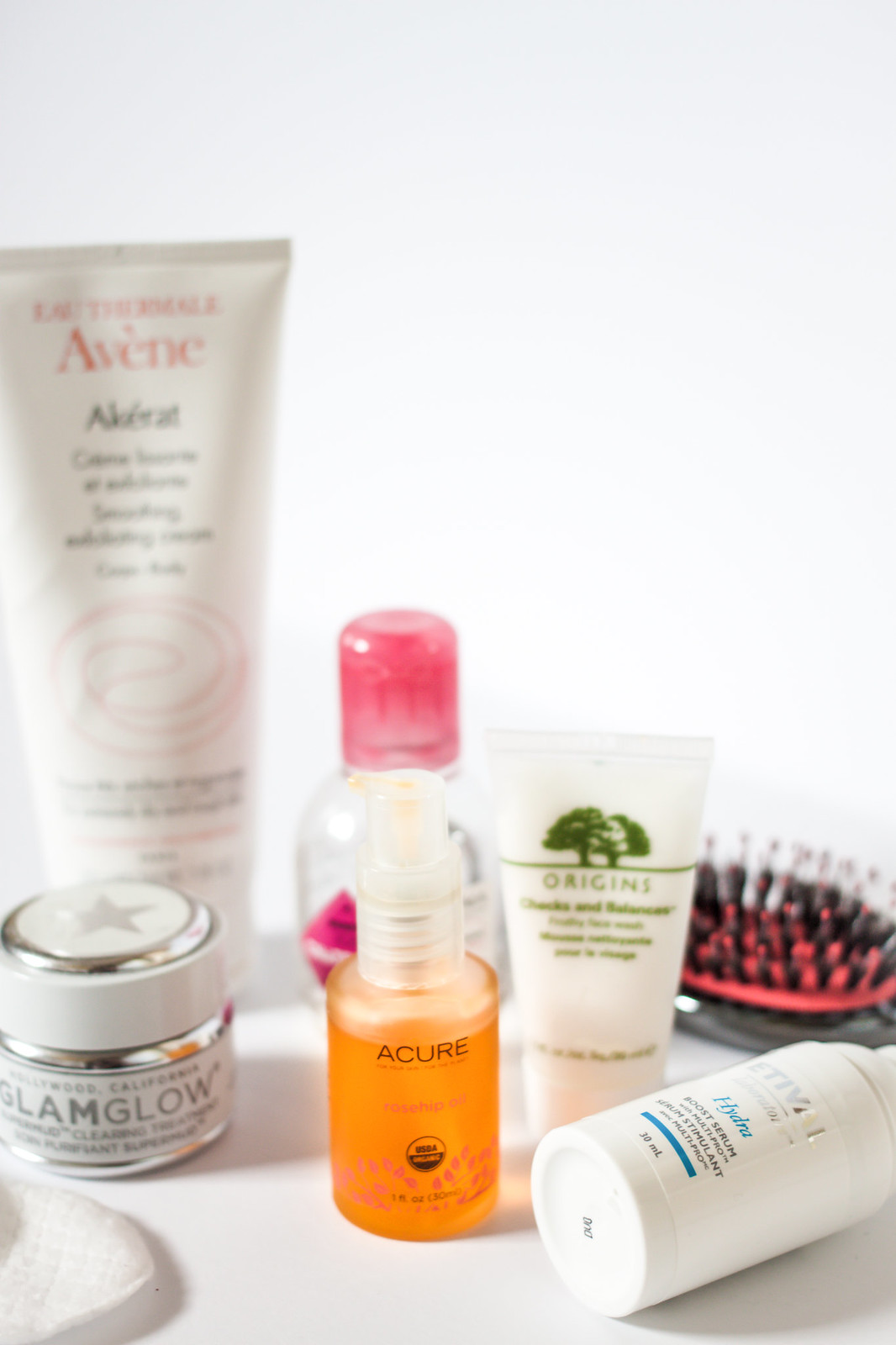The indoor color photograph showcases a professional product display, resembling an image you'd find in a catalog or online store, featuring beauty and skincare products. The scene is set on a white table with a crisp white background, emphasizing the clean and minimalistic theme. 

Starting from the left:
1. In the left foreground, there's a small jar with a white cap, adorned with a white label that reads "Glam Glow" in grey lettering.
2. Behind the jar, a white tube of cream can be seen. The top of the tube features "Aveeno" written in bold red letters.
3. Moving to the right foreground, there is a small clear plastic bottle, likely holding an ounce or two of liquid. This bottle, equipped with a spray applicator and filled with an orange liquid, is labeled "ACURE" in black lettering.
4. Directly behind the ACURE bottle, a clear bottle with a pink cap is visible. The label of this bottle is obscured by the ACURE bottle in front of it.
5. Slightly right of center and behind the ACURE bottle, a small white tube with "Origins" printed in green letters is arranged.
6. Directly behind the white tube, the head of a black brush with pristine black bristles is displayed, appearing brand new.
7. In the far right corner, a white plastic bottle, approximately three ounces in capacity, lies on its side, pointing diagonally. Only the bottom of the bottle is visible as the top extends out of frame to the right.

The foreground objects are much clearer and in sharp focus, while the background objects are slightly blurred, adding depth to the composition. No additional text or print is visible beyond the product labels.